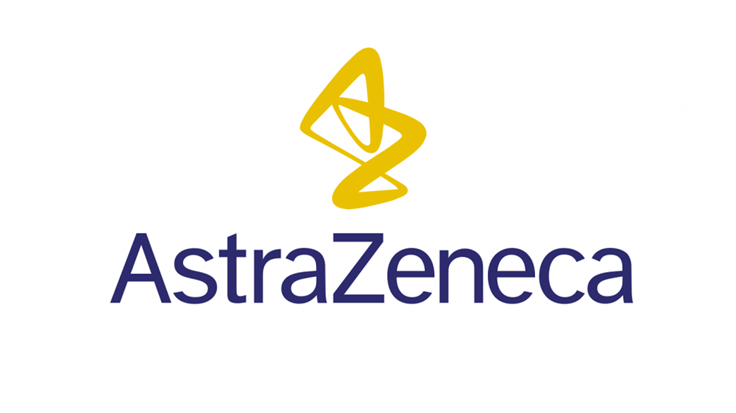The image is a logo set against a white background, featuring prominently the text "AstraZeneca" in a blue-purple color with a capital 'A' and a capital 'Z'. The font appears plain and unremarkable. Above the text, there is a distinct mustard-colored design that intertwines an 'A' and a 'Z'. This design starts with a squiggly line forming the 'A', which seamlessly transitions into the 'Z' as the line wraps around to touch the left side of the 'A'. The entire design resembles a bold, abstract scribble, varying in thickness, and can be likened to a continuous, fluid stroke akin to a stylized racetrack.